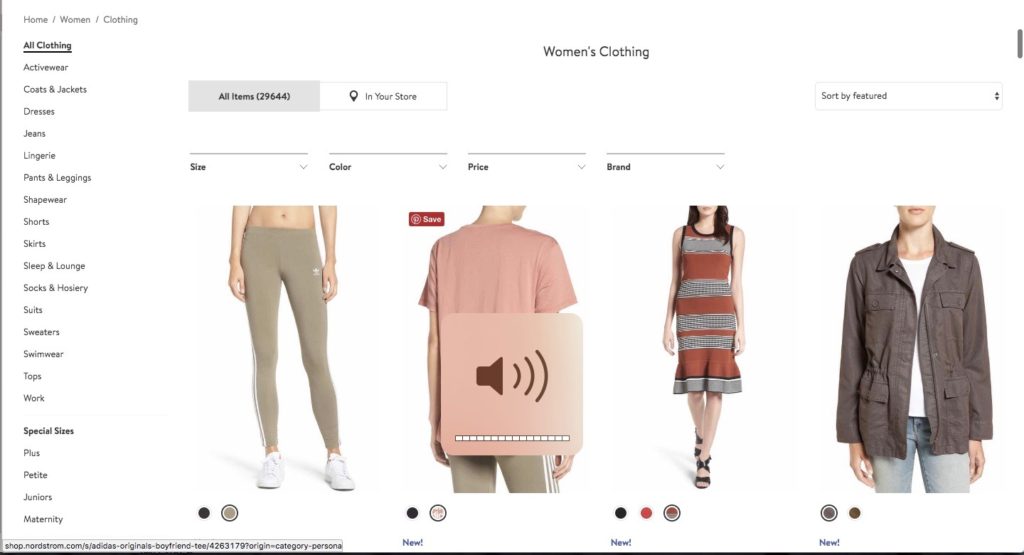The image captures the screen of a woman's apparel website, displayed on what appears to be an Apple device, likely an iPad given the visible volume icon in the center of the screen, turned all the way down. The website header prominently features the text "Women's Clothing" in bold, smaller font at the top center. Below this header, the main content area showcases four distinct images of women's wear: from left to right, a woman in bare pants, a short-sleeve t-shirt, a dress, and a coat. On the left side of the screen, there is a navigation menu with "All Clothing" clearly listed at the very top, providing users with easy access to browse the complete collection.